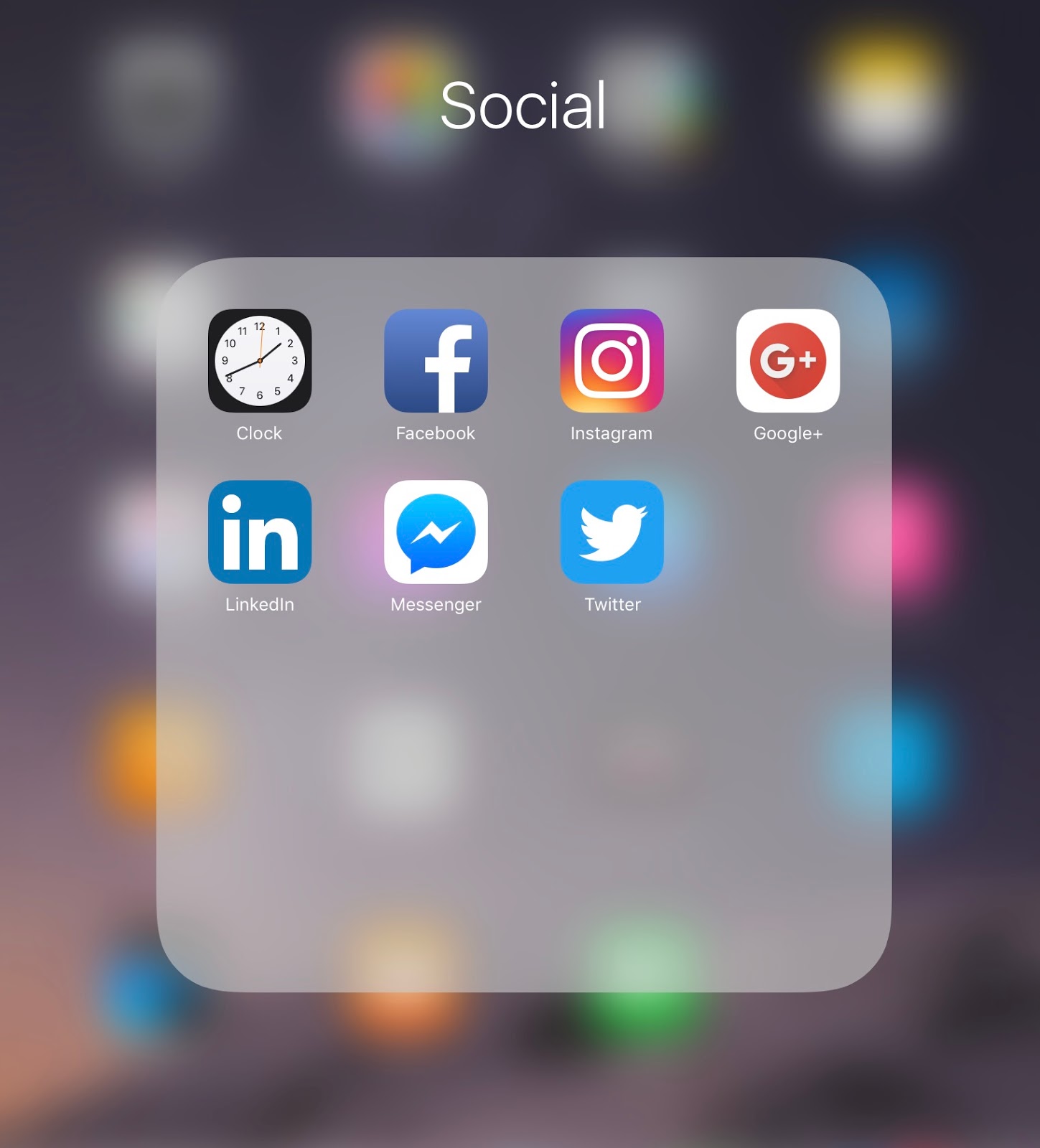The image, captured on an iPhone and magnified for detail, focuses on a section displaying various app icons. The icons appear heavily blurred and muted, with their specific details obscured, though the colors are still distinguishable. Notable colors include orange, green, blue, hot pink, and a mix of multiple shades, as well as black and white.

Amidst the vaguely visible icons, a prominent gray pop-up with rounded edges is centered in the image, further detailing the app icons it overlays. The app icons, listed in order from left to right, include:

1. **Clock**: Depicted as a clock face.
2. **Facebook**: A blue background with a white 'F'.
3. **Instagram**: A multicolored gradient (purple, yellow, red) with a white square and circle in the center.
4. **Google+**: Shown as a white 'G' and plus sign on a red background.
5. **LinkedIn**: Blue with white 'IN'.
6. **Messenger**: White background with a blue chat bubble.
7. **Twitter**: Blue background featuring a white bird icon.

Each icon retains its iconic color scheme and partial visibility, aiding in their identification despite the overall blur and muted presentation.